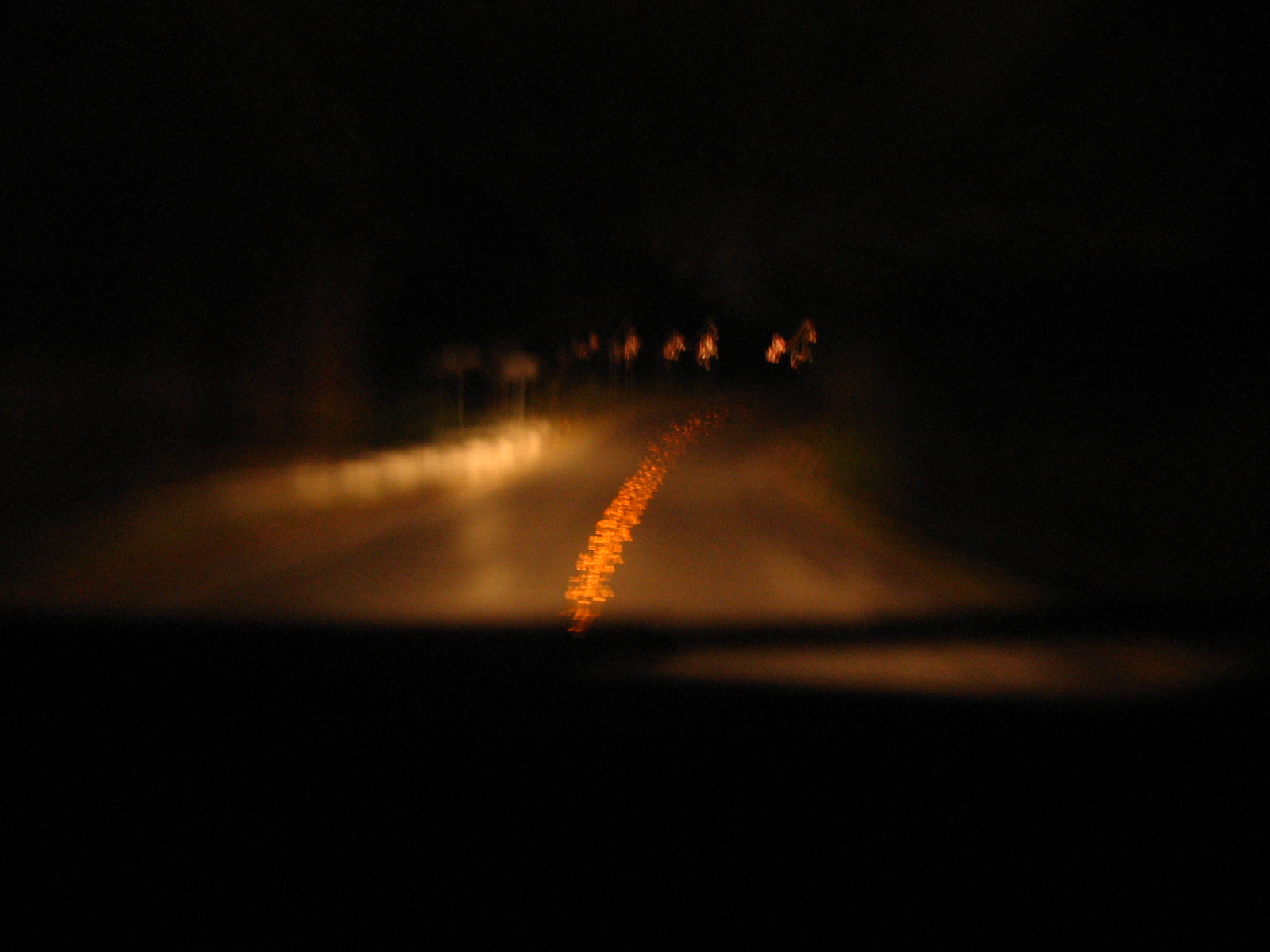This color photograph, taken at night with very dim lighting, captures a view from the passenger side of a car, looking directly out of the windshield onto the road ahead. At the bottom of the image, the dashboard is silhouetted in darkness, with a single windshield wiper blade faintly visible. The road itself has a golden shimmer, possibly due to special effects or a filter applied by the photographer. A distinct yellow line runs down the center of the road, appearing speckled and intriguing in the low light. In the distance, there are traffic lights visible, casting a subdued glow, and on the left side of the road, hints of the oncoming traffic lane can be seen, further adding to the scene's atmospheric depth.